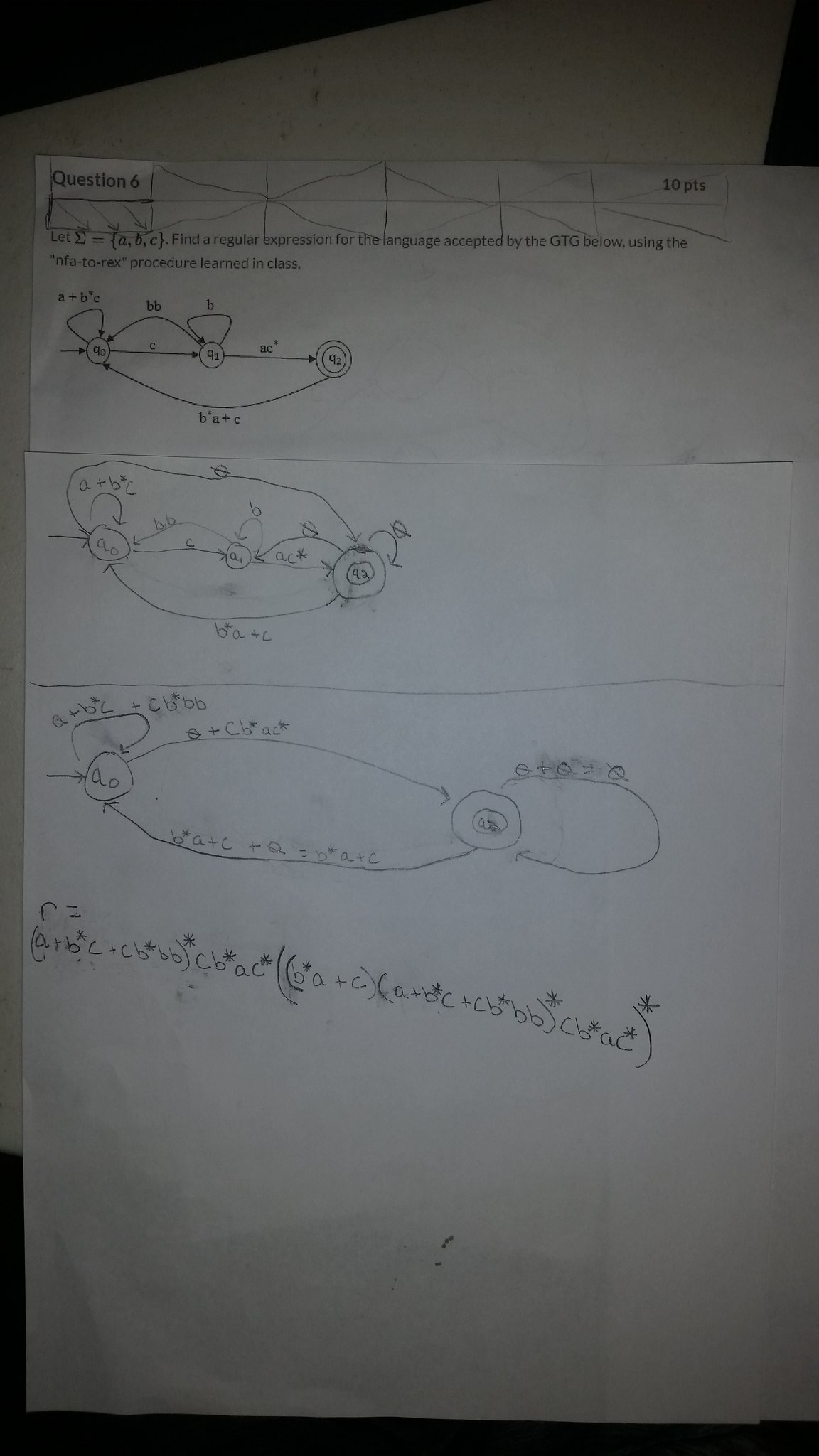This image features a detailed photograph of a test question displayed on a piece of paper, set against a white tabletop background. The bottom edge of the image reveals a dark black area, likely representing the edge of the table, as nothing else is visible below. 

At the top of the paper, "Question 6" is prominently written with "10 points" noted in the upper right-hand corner. The question begins with the statement: "Let epsilon equal [A, B, C]. Find a regular expression for the language accepted by the GTG below, using the NFA to REX procedure learned in class."

Below the textual prompt, a segmented diagram is displayed, possibly representing a generalized transition graph (GTG). The equation depicted reads "A + B * C," and various nodes and arrows are illustrated with corresponding labels:
- Node Q0 has an arrow looping back to itself labeled "A + B * C."
- Node Q2 has an arrow looping back to Q0 labeled "B * (A + C)."
- Node Q1, positioned between Q0 and Q2, features a loop back to itself labeled "B" and an arrow back to Q0 labeled "BB."
- The arrow directing from Q0 to Q1 is labeled "C."
- The arrow from Q1 to Q2 is labeled "AC."

Underneath the GTG, the solved equations are presented, showing the reconfiguration of the initial equation with arrows and symbols indicating transitions. More specifically:
- Q0 to Q2 includes an arrow with a circle and line through it, and the equation is redrawn with an arrow from Q2 back to itself.
- Q2 to Q1 also shows a similar icon.

Subsequent to this illustration, a complex expression is detailed, broken down into algebraic manipulations iterated through several stages:
"A + B * C + C * CB * BB" 
and
"(Q0 to Q2) = 0/ + CB * AC * 0 / = 0 or R = ((A + B * C) + C * (CB * BB)*) * (CB * AC) * ((B * (A + C)) + (A + B* C) + CB* BB)** (CB * AC)** (B* (A + C)) (A + B** C + CB* BB)** (CB* AC)** ."

This extensive series of symbols and variables represents the systematic solution to the problem formulated through the regular expression derived from the NFA to REX process taught in class.